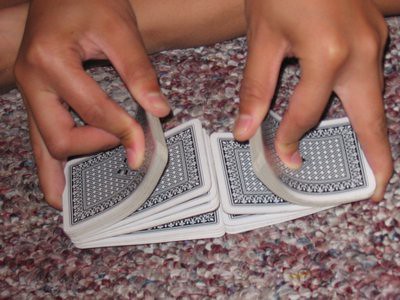In the image, a person appears to be sitting cross-legged on the floor, which is covered with a dark brown and gray short nap carpet. The shin of one leg, noticeably bare, extends diagonally from the top left to the upper right corner of the frame. 

The focal point is a deck of cards with white edges and a gray checkered or speckled background, split into two halves. The left half and the right half of the deck are being manipulated by two hands—one entering from the top left and the other from the top right. Both hands grip the edges of the cards while pressing down in the center with their thumbs, illustrating a vigorous shuffling motion. The cards are bent at a severe angle as they intermingle along the center line.

Notably, the index finger of the left hand appears almost double-jointed, bending backward more extremely than the index finger of the right hand. Additionally, the tip of the left index finger seems disproportionately longer than the tip of the right index finger, adding an intriguing asymmetry to the image.